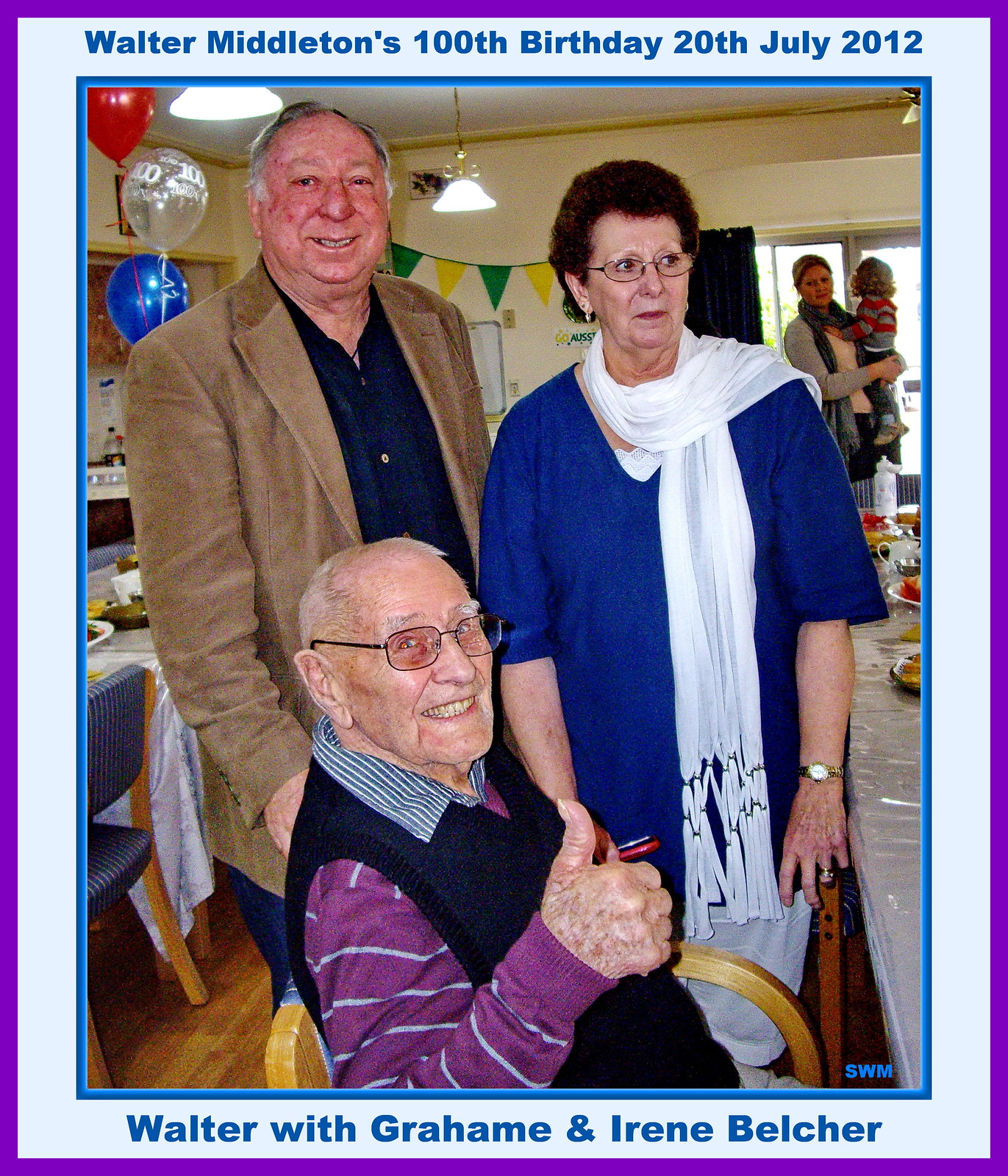The photograph captures a moment indoors at Walter Middleton's 100th birthday celebration on the 20th of July, 2012, as indicated by the blue print on the top white border of the image, which is framed by purple, white, and blue borders. Seated in the center is Walter Middleton, radiating joy with a big smile and a thumbs-up gesture, dressed in a purple shirt layered over a blue shirt and topped with a blue vest. To Walter's left stands Graham Belcher, beaming at the camera in a blue shirt and tan jacket. On Walter's right is Irene Belcher, wearing a blue dress with a white scarf, looking slightly off-camera. The background reveals a festive atmosphere with balloons, banners, and a table adorned with food, suggesting a lively birthday celebration. Also visible is a woman holding a child and various light fixtures, adding to the warm, celebratory ambiance. The bottom white border in blue text identifies the people: "Walter with Graham and Irene Belcher."